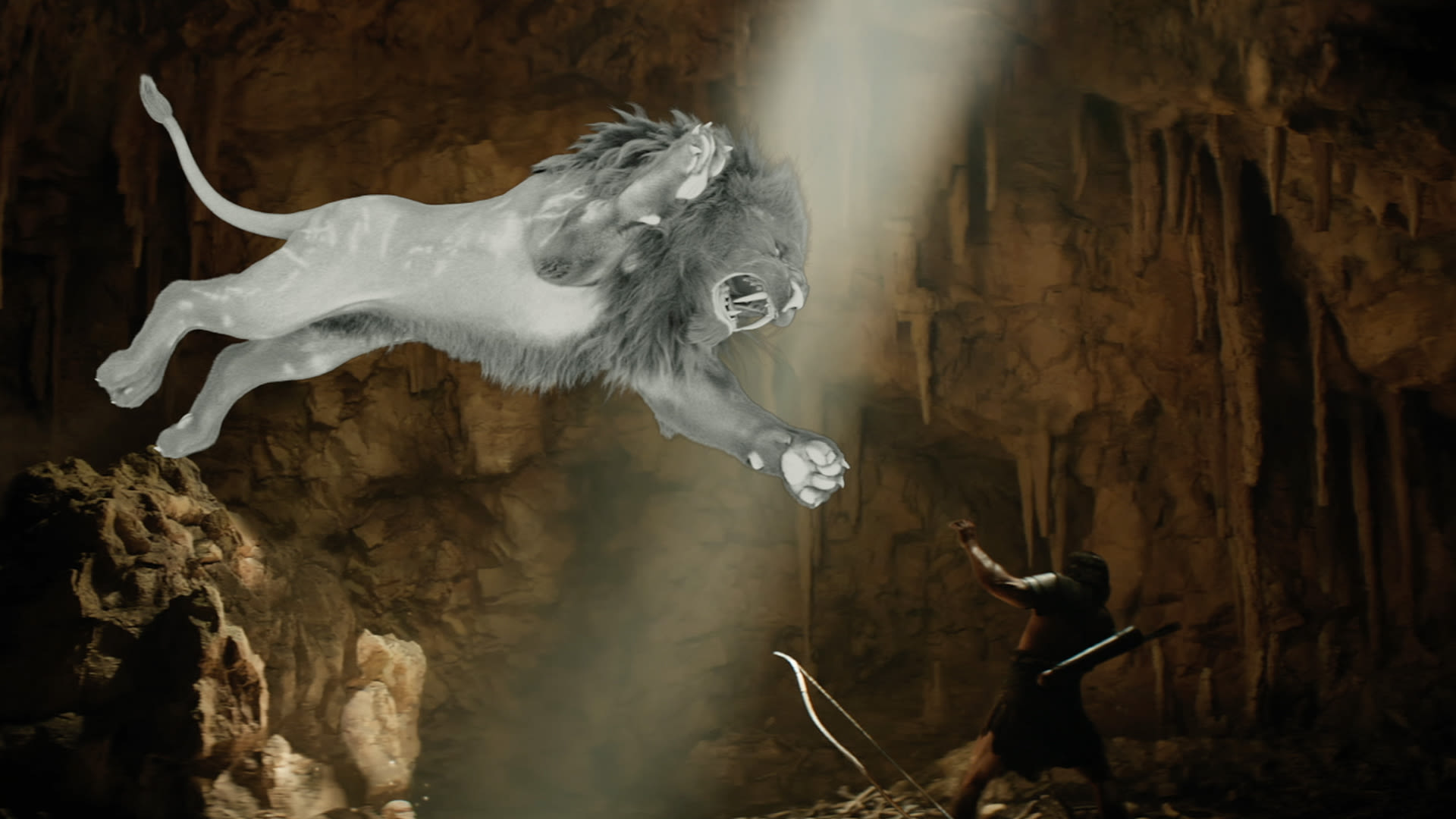The image is an artistic rendering, likely created with advanced digital techniques such as 3D rendering or Photoshop. It depicts a dramatic and intense scene set inside a cave adorned with dark brown and black stalactites hanging from the ceiling. On the left half of the image, a fierce, gray lion with visible scars on its hind flanks and body is mid-leap, frozen in a powerful and aggressive pose as it lunges toward the right side of the frame. The lion, strikingly rendered in monochrome shades of gray, contrasts sharply with the rest of the composition.

To the right, a warrior is seen cowering and raising his left arm defensively. The warrior has dark hair and is clad in a brown loincloth; his chiseled, shirtless torso is exposed. His face and body language speak volumes about the imminent danger he faces. In the scene's foreground, the warrior appears to have just dropped a bow, now lying at his feet alongside a nearly empty quiver on his back and a sickle-like weapon in his hand.

A single shaft of light cuts through the otherwise dark cave, illuminating the intense encounter between the lion and the warrior, adding a dramatic flair to this captivating scene.